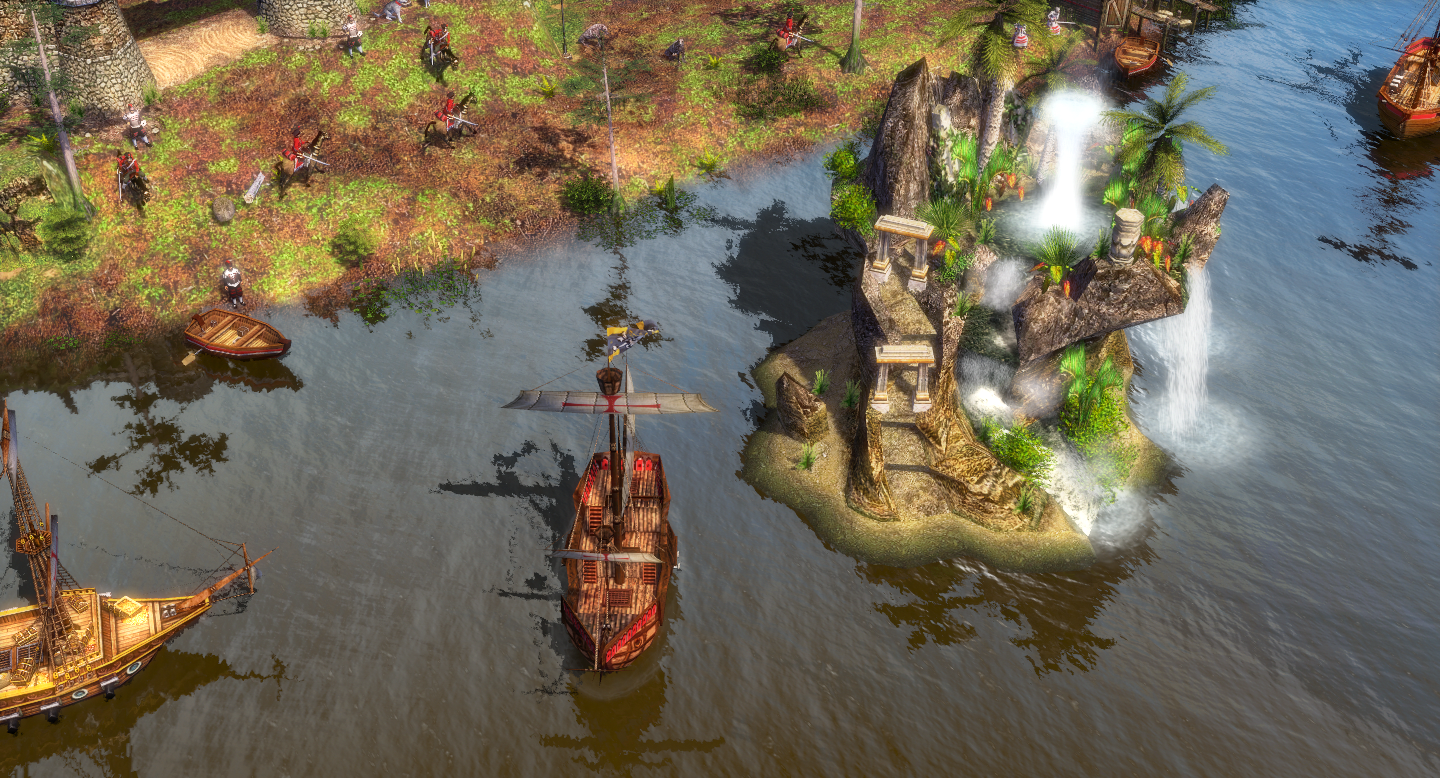The image is a vividly stylized, animated screenshot from a video game, likely set in a medieval or fantasy world, characterized by bright colors and intricate details. In the lower right section, a small island emerges from the dark sea, featuring a rock-formed structure, verdant plants, and cascading waterfalls that suggest a fountain-like formation. Surrounding the island, several wooden ships of various brown hues, with at least one distinctly red and another yellowish, float in the water. The top left corner transitions into a shoreline with grass and soil, where soldiers, possibly from the medieval or early modern era, are seen on horseback dressed in red coats and armed with swords or guns. Nearby, a small rowboat rests on the shore, next to which a lone figure stands, seemingly busy with tasks. The shore area also contains some vegetation and a partially visible brick building, adding to the historical or fantastical ambiance of the scene.